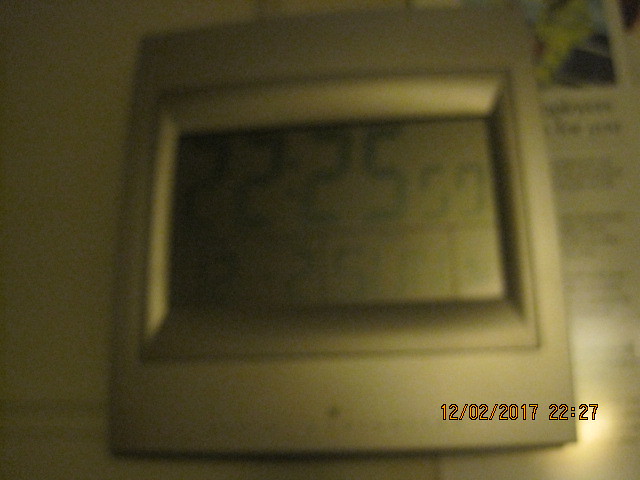The image shows a close-up photograph of a square, silver-colored digital device with an LCD screen, likely a timer or stopwatch, indicating the time 22:25. The device appears old and occupies a significant portion of the photograph (60-75%). The screen is divided by a black line, with larger numbers on the top and smaller, vertically sectioned numbers on the bottom. The background of the image is blurry, featuring a white pamphlet with blue text and an image above the text, as well as a partially visible poster with text and a yellow character. The photo has a timestamp in the bottom right corner, dated February 12, 2017, at 22:27. The lighting is uneven, with the bottom right corner well-lit and the top left progressively darker.